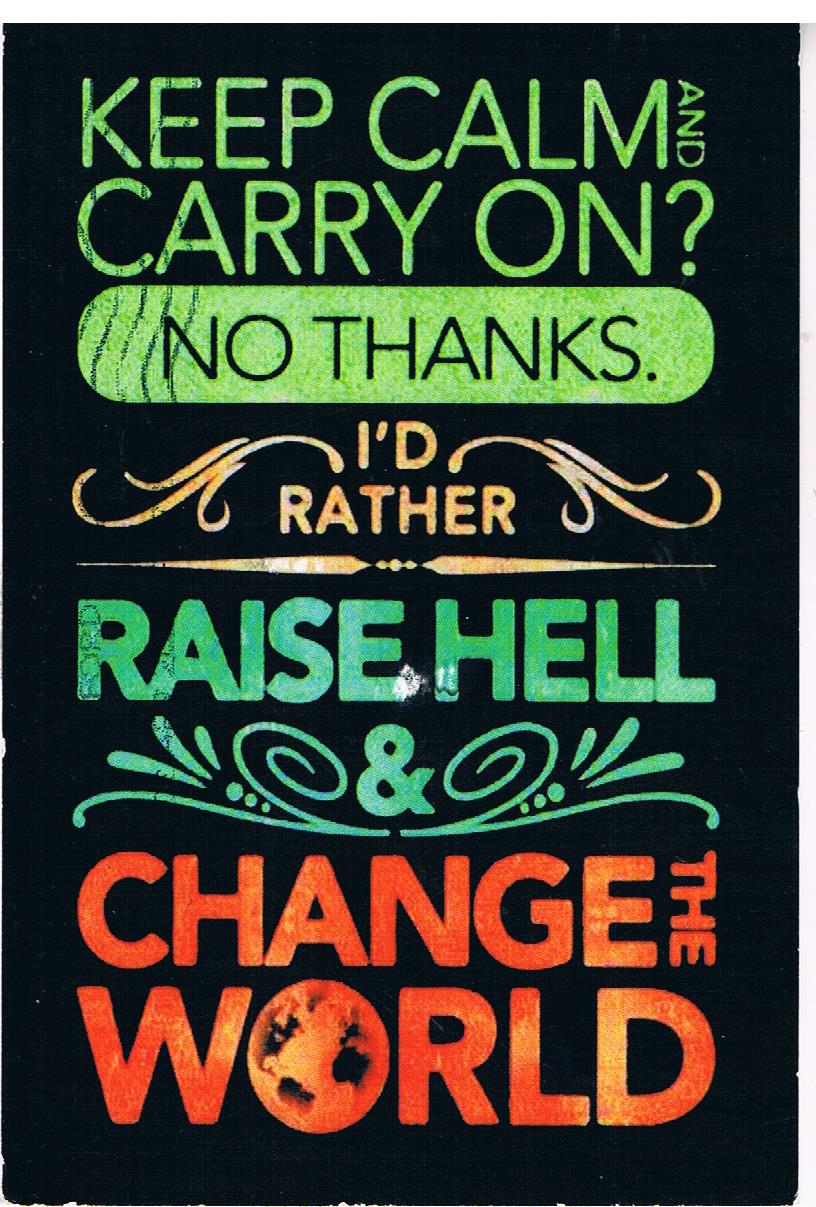The image is a stylized, inspirational poster set against a black background, vertically aligned with various colors of text. At the top, in mottled green font, it reads "KEEP CALM AND CARRY ON?" followed by "NO, THANKS" in yellow. Below that, in orange font, it states "I'D RATHER," adorned with curly, swirly floral designs extending horizontally from both sides. Underneath, in large green uppercase letters, it declares "RAISE HELL," followed by an ornate green ampersand symbol with more floral-like patterns around it. The final line, in green uppercase font, says "CHANGE THE WORLD," with the letter 'O' in "WORLD" designed to resemble a globe, featuring crack-like lines that outline continents.